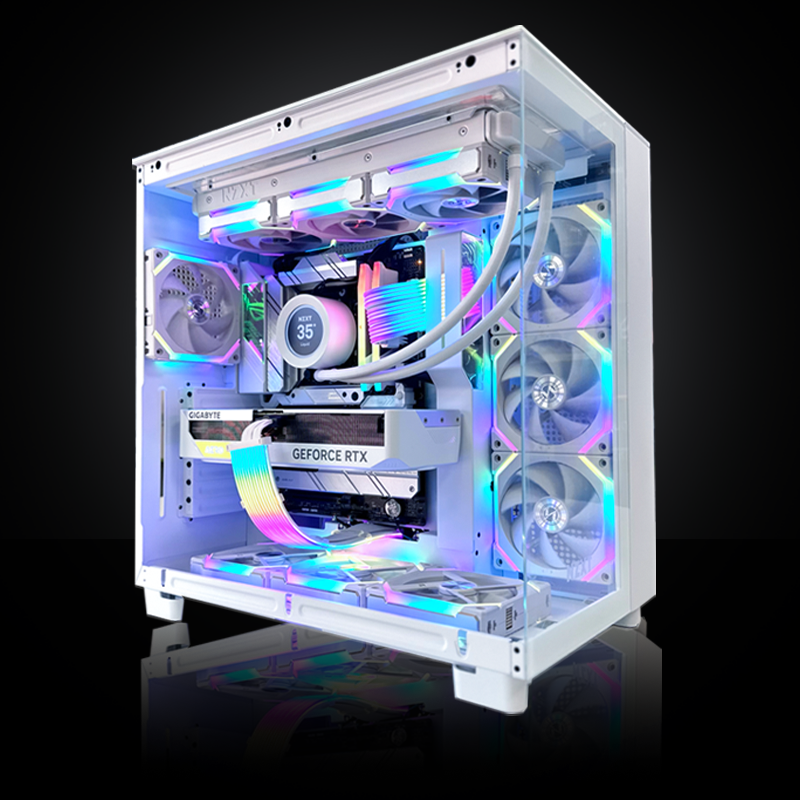The image showcases the intricate interior of a high-end computer tower set against an all-black background. Visible through a clear glass panel, the machine's interior is illuminated by an array of vibrant colors—blue, yellow, and pink— highlighting its advanced components. Prominently featured are three vertically arranged fans on the right side, three horizontally aligned fans at the top, another three at the bottom, and a single fan on the left side, all glowing in neon blue, aqua, purple, and pink hues. Notable branding includes 'GeForce RTX' emblazoned on a lower component and 'Gigabyte' inscribed in the top-left corner of the machine. Several colorful fiber cables—blue, yellow, and pink—snake through the setup, adding to the aesthetic complexity. The reflective surface beneath the tower enhances the visual appeal, casting a subtle mirror image of the machine.